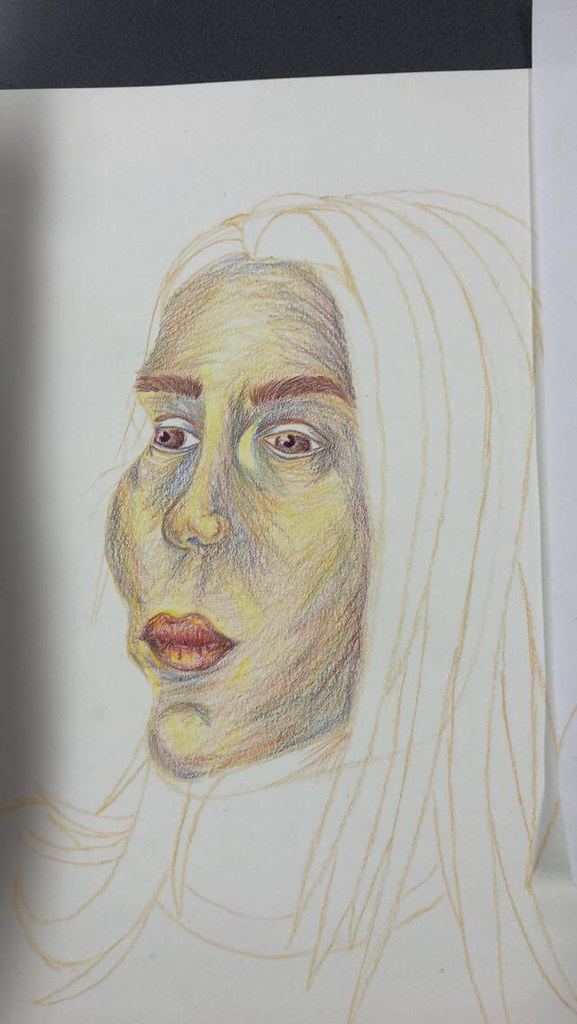This vertical photograph captures a relatively detailed sketch on a white piece of paper, bordered at the top by a black edge. The piece appears to be created using pencils or crayons and is unfinished. The sketch portrays a woman from the shoulders up, with exaggerated and misaligned facial features in a caricature-like style. The face is richly colored and shaded with hues of yellow, red, black, purple, blue, and brown, enhancing an eerie quality. Her full lips are distinctly red, while her eyes, shaded in greenish-brown with white eyelids, sit under thick brown eyebrows. Despite her hair being outlined and described as long and shoulder-length, it remains uncolored, cascading down in a parted style. The figure wears a turtleneck shirt, and the face is tilted to the right, presenting a view primarily of the left side at a 45-degree angle. The chest and hairline are drawn in a light brown tan color, emphasizing the unfinished state of the artwork. The entire sheet rests on a visible white surface beneath it.